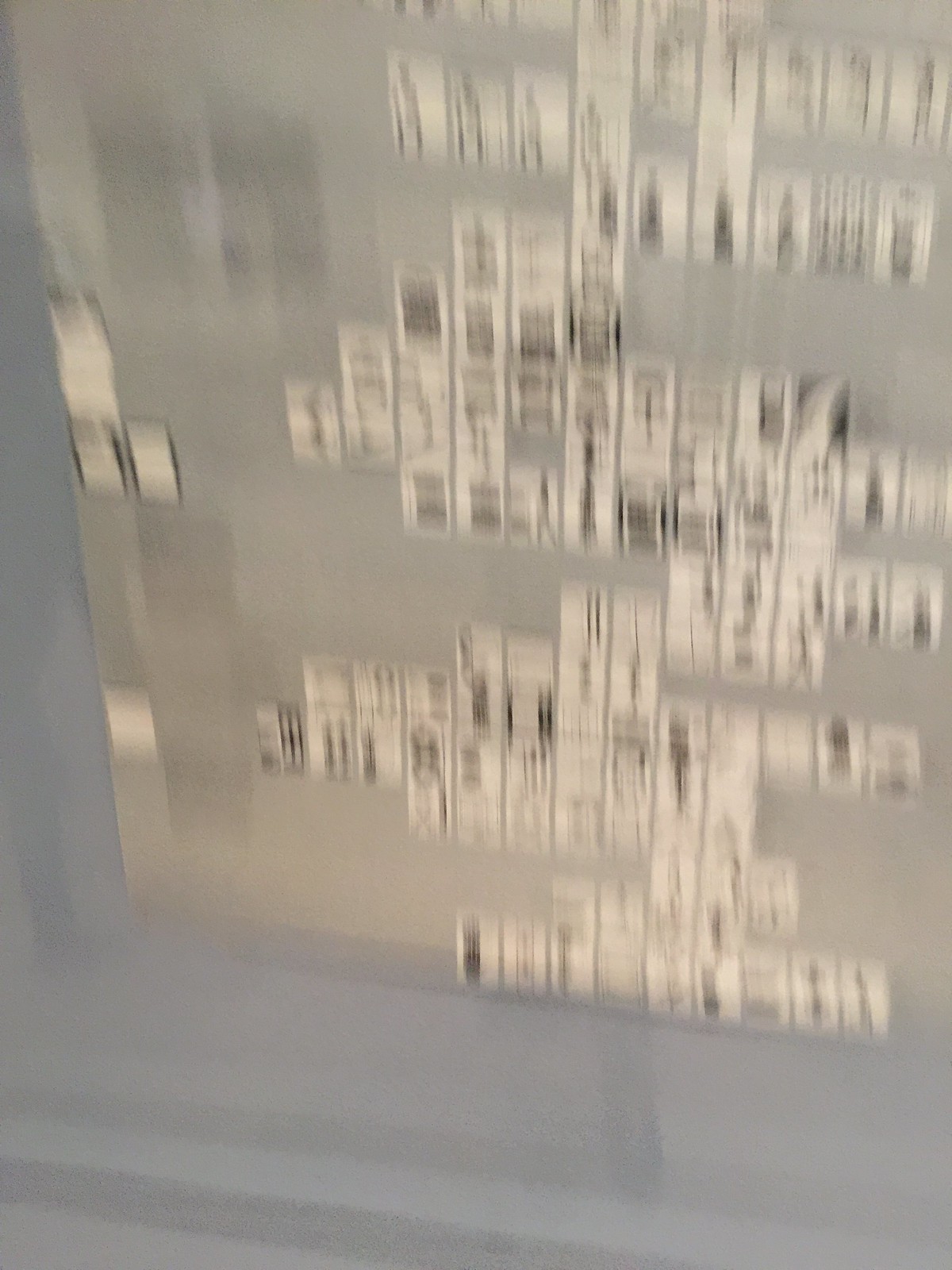This image captures a highly blurred and out-of-focus scene featuring a large rectangular gray poster adorned with numerous small square black-and-white photos or drawings. The poster is mounted on a light blue wall, creating a soft color contrast. Due to the lack of focus, no specific details of the images on the poster can be discerned, only the general shapes and colors. In the bottom left corner, the wall appears to have a darker blue border or a slight protrusion, adding a subtle variation to the otherwise uniform background.